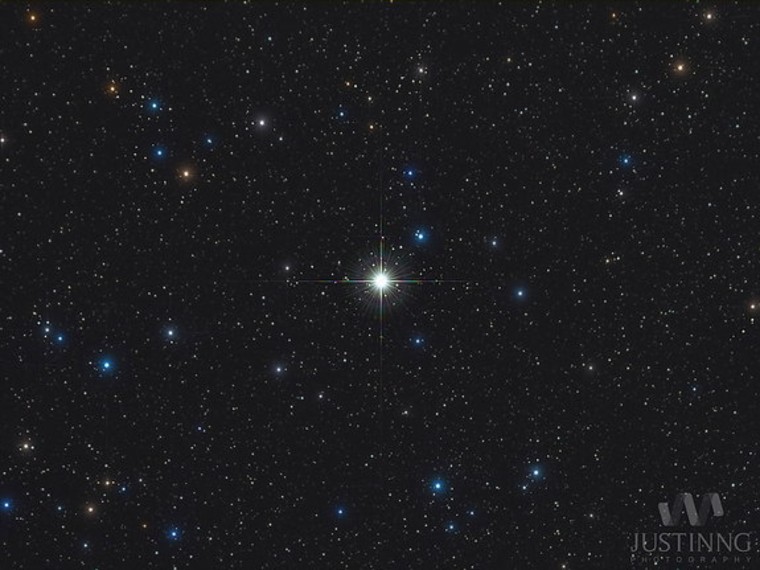This photograph features a captivating view of the night sky, presenting the vast black expanse of space adorned with numerous multicolored stars. The stars vary in shades, including tiny white, yellow, red, orange, and blue dots scattered across the image. The central focal point is a distinctly bright star emitting a prominent halo and light beams that create a cross-like twinkle effect. This star exhibits a diamond-like appearance with subtle hints of rainbow colors. Additionally, some larger blue and orange dots glow faintly, adding depth to the celestial scene. A watermark resides at the bottom right corner of the photograph, featuring a wavy line logo followed by "JUSTINNG" and the word "photography" beneath it in gray lettering.